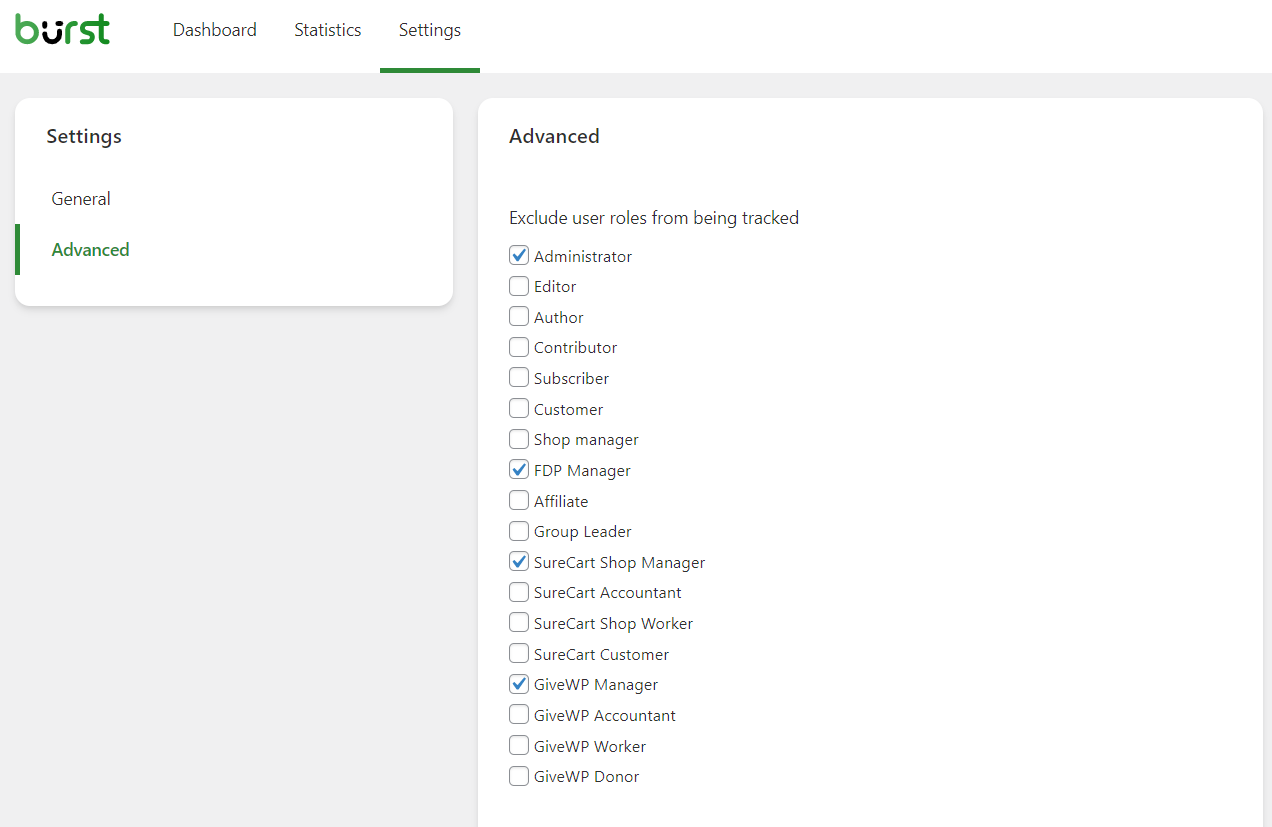The image depicts a user interface with a clean, white background interspersed with sections featuring a light gray background. In the top left corner, the word "Burst" is prominently displayed; the letters 'B', 'R', 'S', and 'T' are green, while the 'U' remains black. The interface includes tabs labeled "Dashboard," "Statistics," and "Settings"—the latter being underlined in green to indicate that it is currently selected.

Below, against the light gray background, is a medium-sized white rectangle with the title "Settings" in black text. Within this section, there are two sub-tabs: "General" in black text and "Advanced" in green text, with the latter additionally highlighted by a green line, signifying it as the active tab.

Expanding from this, there is a larger white, squarish area labeled "Advanced" in black text. Underneath, the section "Exclude User Roles From Being Tracked" is listed, containing various user roles each accompanied by a checkbox. The roles are as follows: "Administrator" (checked), "Editor," "Author," "Contributor," "Subscriber," "Customer," "Shop Manager," "FDP Manager" (checked), "Affiliate," "Group Leader," "Sure Cart Shop Manager" (checked), "Sure Cart Accountant," "Sure Cart Shop Worker," "Sure Cart Customer," "Give WP Manager" (checked), "Give WP Accountant," "Give WP Worker," and "Give WP Donor."